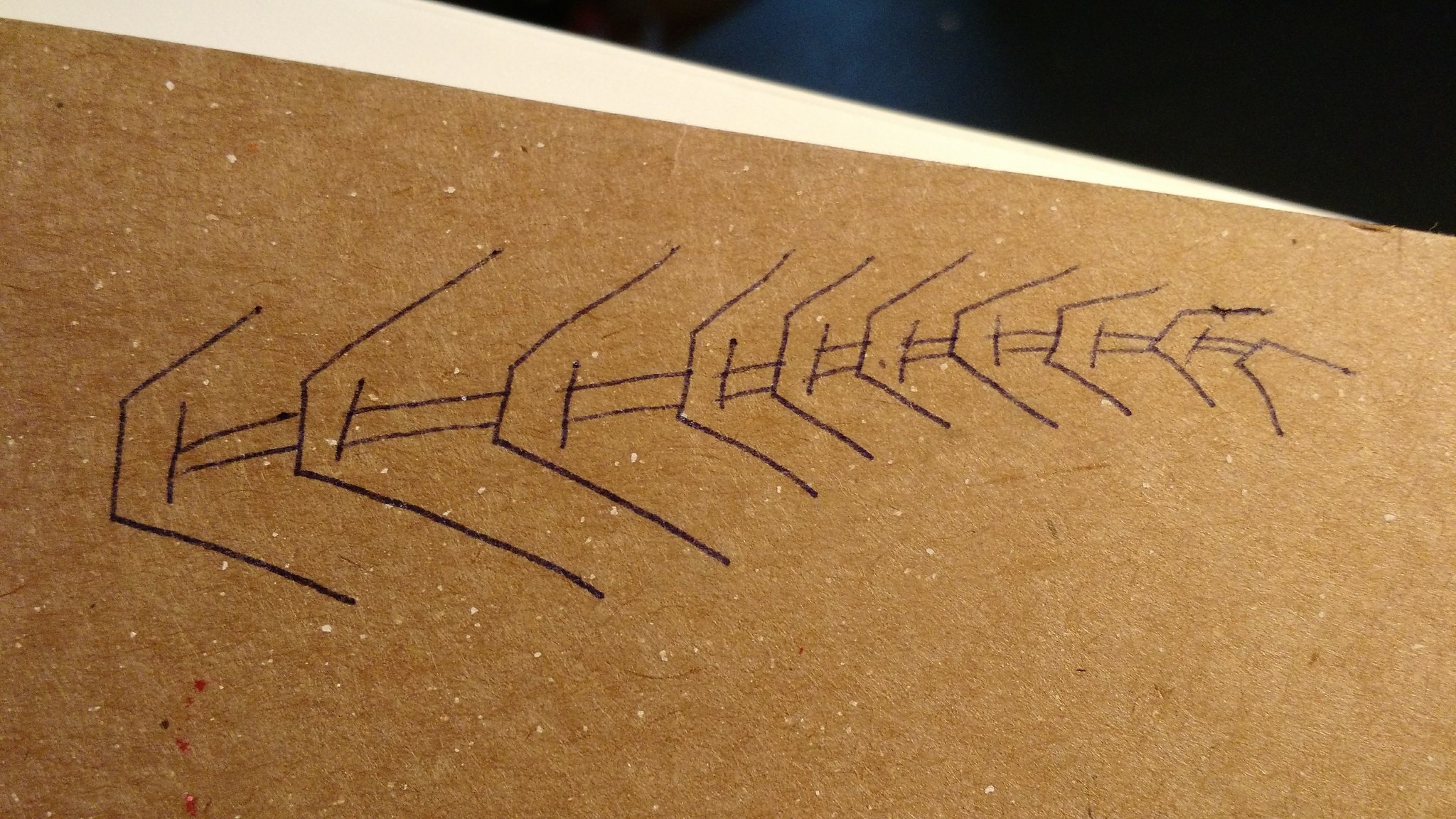The image depicts a piece of brown, recycled cardboard that resembles the back cover of a notebook. The surface of the cardboard is peppered with tiny white specks, giving it a somewhat uneven texture. On the cardboard, there are black pen marks arranged in a distinctive pattern: a series of straight lines intersected by pairs of perpendicular lines. This pattern repeats nine times from left to right, with each successive figure decreasing in size. Below the cardboard, a sliver of a white surface is visible, hinting at the background on which the cardboard rests. In the top right corner of the image, there is a dark, indistinct mark. Apart from these line drawings, the image contains no text or additional distinguishing features.